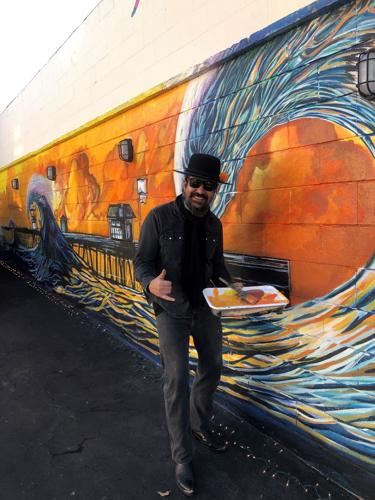The photograph features a bearded artist, dressed entirely in black—wearing a black hat with a circular brim, dark sunglasses, a long-sleeve black jacket, black shoes, and gray pants. He stands on black asphalt with a cinder block wall in the background. In his right hand, he makes a gesture with his thumb up and pinky extended, while in his left hand, he holds a white palette with visible orange and yellow paint. Behind him, a vibrant mural covers most of the wall, depicting a series of large, curling waves reflecting the hues of a bright orange sunset. These waves showcase facets of blue, yellow, orange, and white, creating a stained glass-like effect. The mural also includes a dock with small buildings. The sky above the waves is a meld of red, orange, and yellow colors. The upper part of the wall is left unpainted, revealing its white surface.